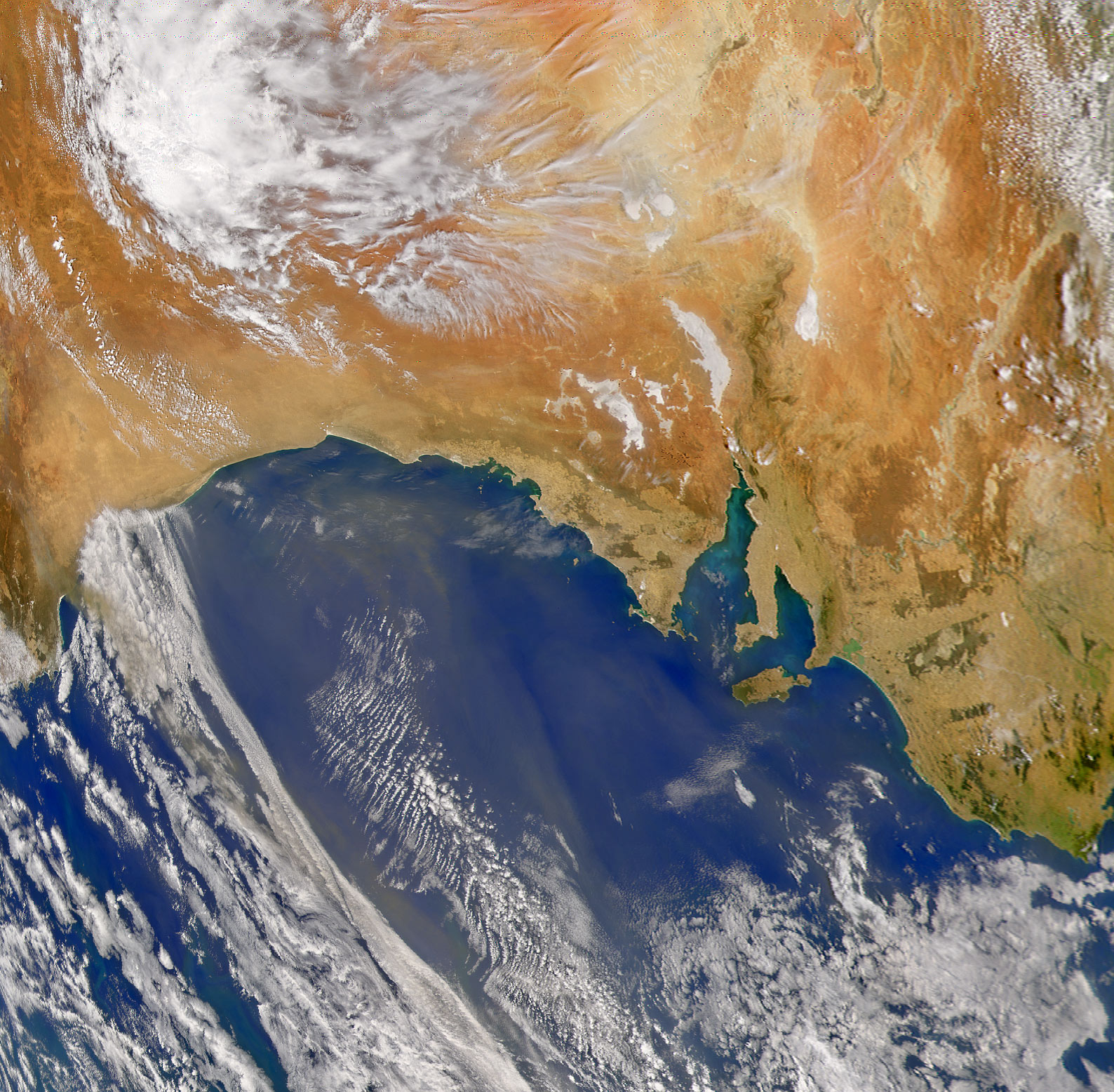This detailed aerial image provides a mesmerizing view of Earth's surface, with a clear division between a landmass and a body of water. The upper portion of the image showcases a diverse landmass in hues of light green, light brown, reddish, and golden brown, interspersed with streaks of white clouds. Clouds form noticeably in the upper left corner and continue to scatter across to the right, where two smaller clouds hover above the landmass, culminating in a large cluster on the far right edge. Meanwhile, the bottom half of the image is dominated by a vibrant blue expanse of water, likely the ocean, featuring spatterings of bright white clouds. These clouds are most dense on the left side, almost completely covering it, then give way to an open patch of clear blue water towards the center-right. Beneath the main landmass sits a small island in the water, adding an intriguing detail to the scene. Overall, the image offers a dynamic contrast of terrestrial and aquatic elements, accentuated by the varying intensity of cloud cover.